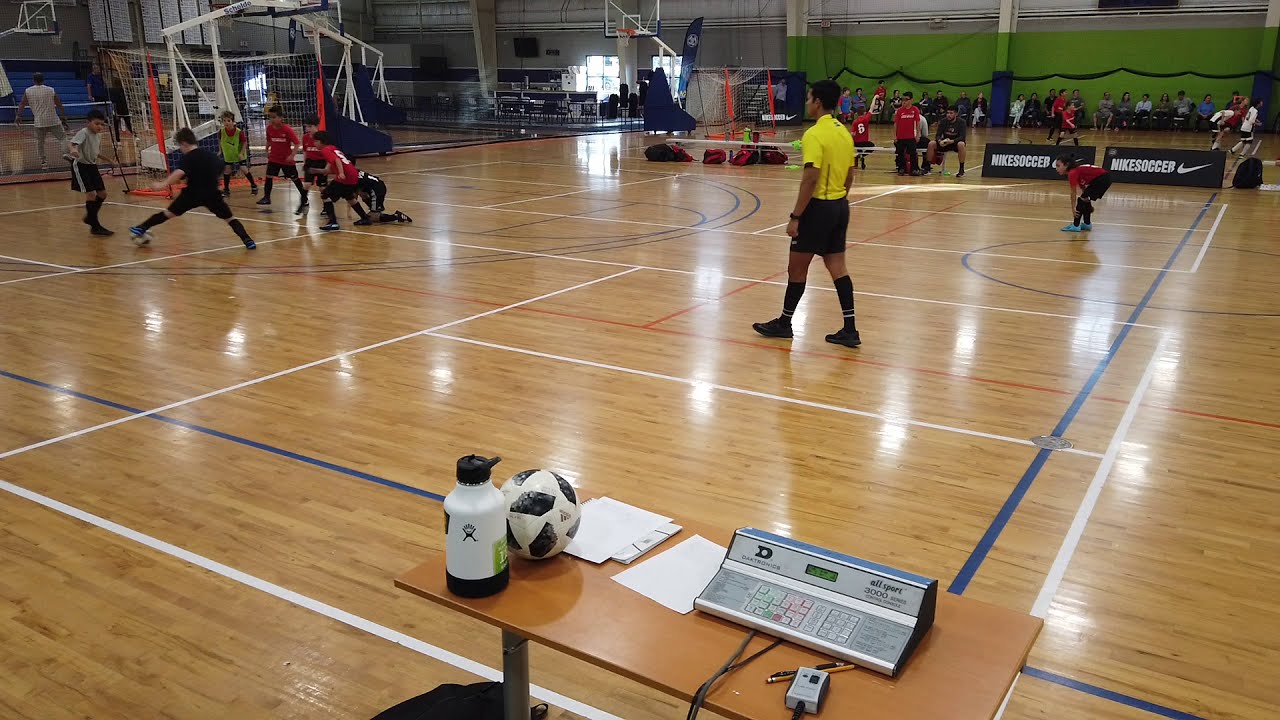An image captured from a slightly elevated position, approximately six feet off the ground, showcases an indoor gymnasium repurposed for a youth soccer practice. The light wood floor, originally a basketball court, has been taped off for soccer, evident from the distinct lines and a visible goal with a net in the background. At the bottom of the photo, a table holds a soccer ball, a water bottle, and an electronic console with buttons and a small LED display, likely used for scorekeeping. 

Several young boys, possibly around 10 or 11 years old, are seen engaged in the practice. One boy in a black shirt is controlling the ball, while another in gray approaches him, and a few boys in red jerseys are gathered nearby. A coach or referee in a yellow shirt and black pants stands out in the foreground, distinct from the players who wear uniforms suggesting two different teams: red and black. 

In the far distance, a green wall is lined with spectators, most likely parents, seated on bleachers. Above them, banners reading "Nike Soccer" with the iconic Nike swoosh are prominently displayed. The background scene is further populated with children practicing with soccer balls, which solidifies the sporting nature of the gathering.